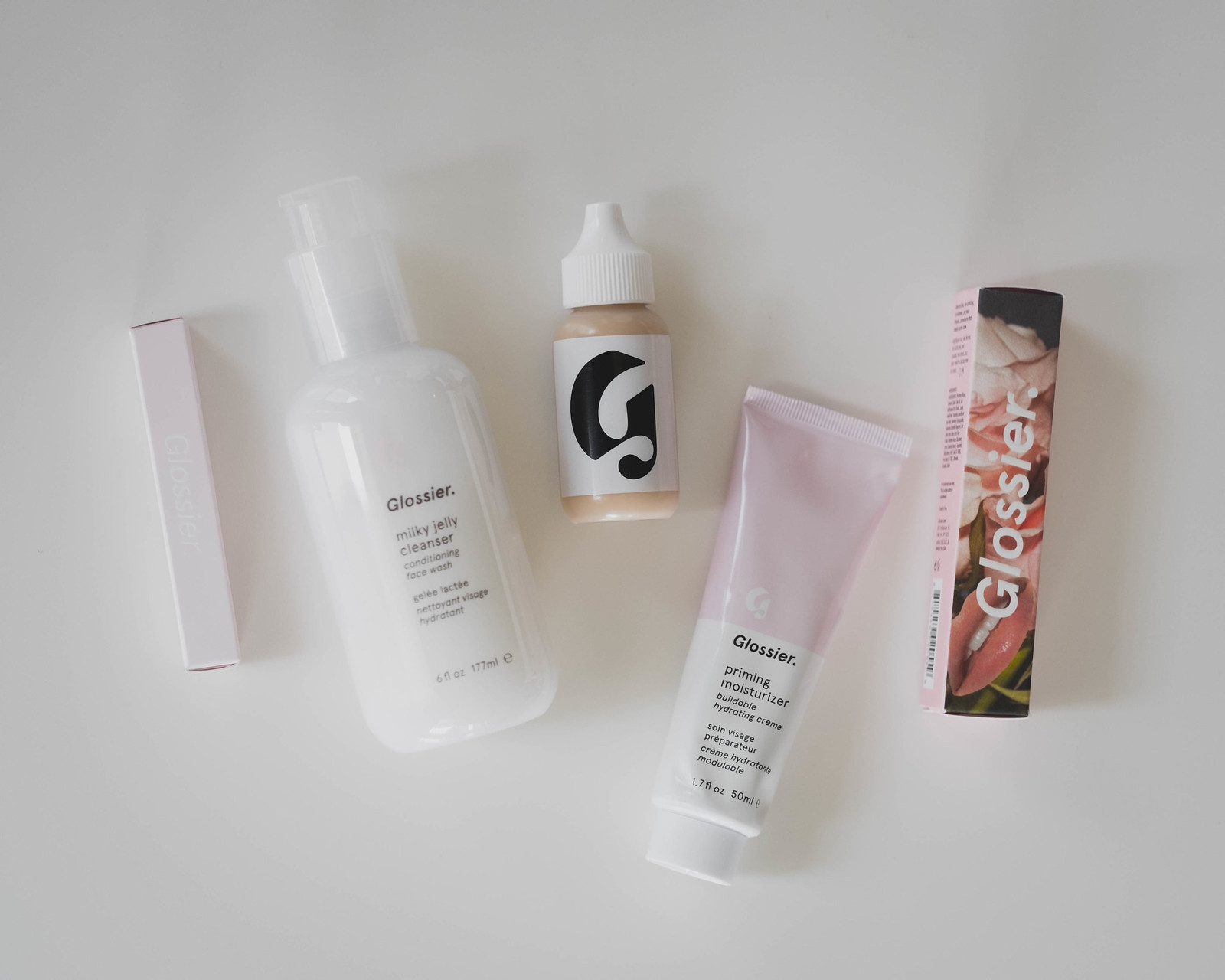Here is a detailed and descriptive caption for the image:

---
This close-up photograph showcases an array of beauty products artfully laid on their sides against a pristine white background. Starting from the left, there's a tall, slender box in a very light pink hue with faint white text that reads "Glossier," though the writing is somewhat difficult to discern. Next to it lies a white bottle with its label facing upward, featuring a clear plastic cap. The black text on the bottle says "Glossier," followed by "Milky Jelly Cleanser Conditioning Face Wash," along with the same information written in French, and the bottle's measurements. Moving right, there’s a bottle resembling an eyedropper with a white cap, characterized by its beige coloration and an elegant black "G" on its white label. Adjacent to this bottle is a tube that tapers from a wider top to a narrower end capped with white. The upper part of the tube is light pink and bordered by a white strip at the bottom. The black text on it reads "Glossier Priming Moisturizer Buildable Hydrating Cream," with corresponding French instructions and measurements listed below. Finally, on the far right, a slender box that looks like it might contain lip gloss is adorned with an illustration of lips, surrounded by roses and leaves. White text, orientated towards the left, spells out "Glossier" at the top of this intricately designed box.

---
This enhanced caption brings clarity and detail to the description of the beauty products in the image.